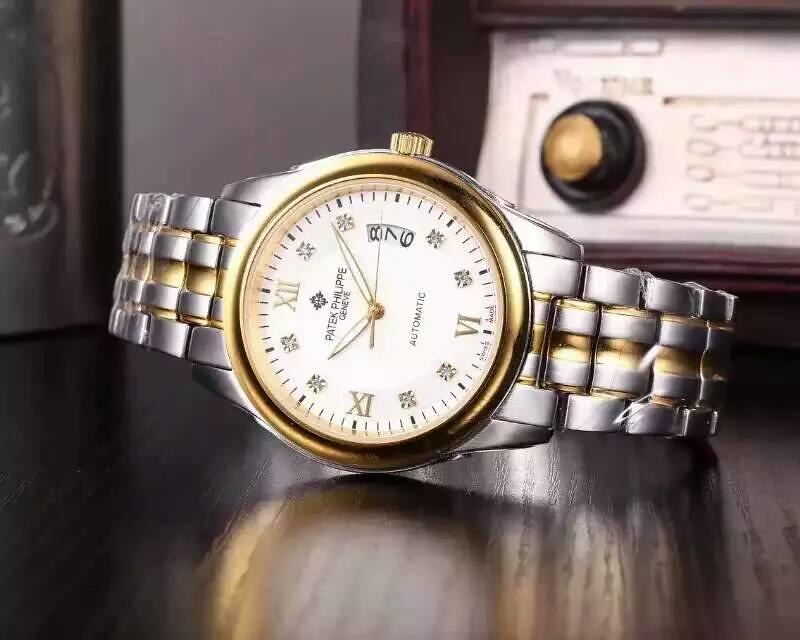In this professional color photograph, a distinguished Patek Philippe automatic wristwatch is prominently featured. The watch, a symbol of luxury, is meticulously rendered in silver with intricate gold accents. Its bracelet is predominantly silver interspersed with three elegant lines of gold, enhancing its sophisticated design. The face of the watch is white, encircled by a golden ring, and elegantly displays gold Roman numerals at the 12, 6, and 9 positions, with the remaining markers suggesting a floral design. The hands are designed as gold bands bound together, accompanied by a slender second hand.

This close-up shot reveals the watch resting on a dark, glossy wooden table, with its polished surface reflecting parts of the watch's white face and gold elements. Behind the watch is an antique analog radio with a dark brown frame and a distinctive white face, featuring a black knob with a gold center on the left side, and faint brown lines and diagrams. The overall background is greyish, blending seamlessly with the reflective wooden surface. Additionally, there are miscellaneous items such as a piece of paper and possibly a glass cup or jar in the periphery, contributing to the composed and classic ambiance of the setting.